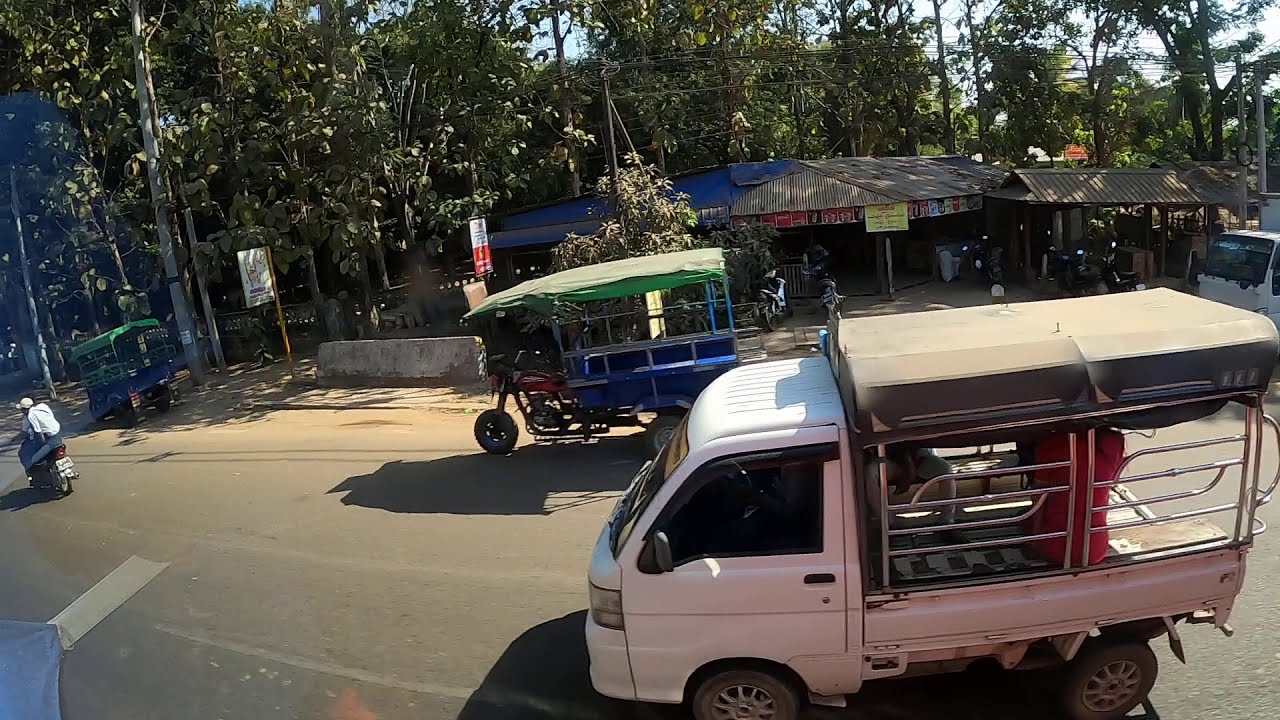This vibrant photo, likely taken in another country, captures a bustling roadway scene from an elevated vantage point, providing a comprehensive vista of the surroundings. Dominating the foreground is a white truck with tinted windows and a silver cage-like structure in the open back, which has bars and cloth sides. Next to it on the other side of the street, there’s a distinctive motorcycle equipped with a red front attachment and an enclosed blue carriage with a green roof, seemingly designed for passenger transport. A man in a white shirt and hat rides a small bike towards the edge of the image, passing a parked motorcycle with a similar blue back and green cloth top. Flanking the street, there are a series of small shacks with dark, metal-looking roofs, which appear to be part of an open-air market, complete with banners and signs visible. The scene is set on a wide roadway under a bright, sunny sky with thick clusters of trees in the background that are densely populated, allowing patches of clear blue sky to peek through.